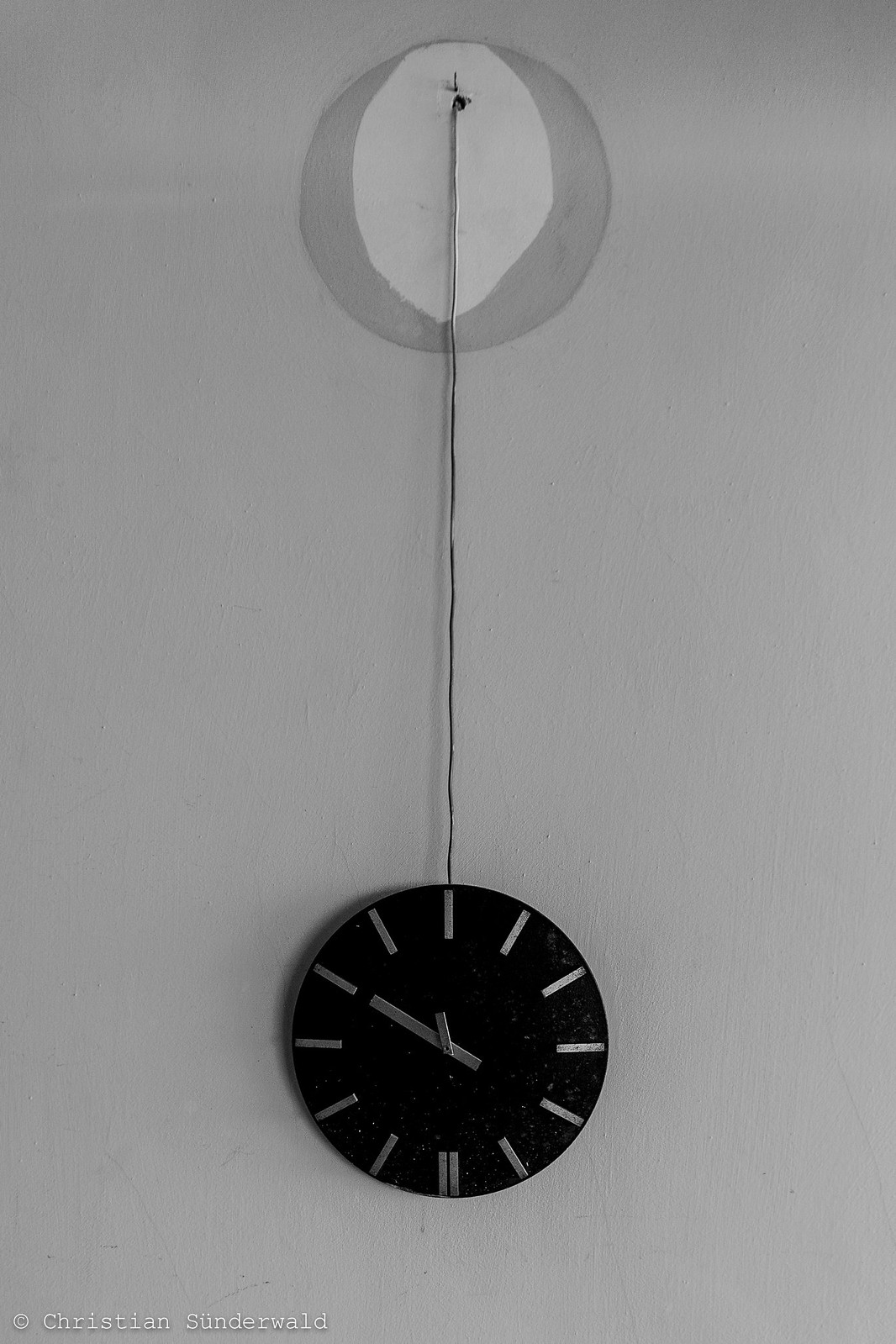The image features a simple yet striking art piece by Christian Sondervold, presented in portrait mode. It shows a black clock hanging from a hook on a gray wall. The wall has two distinct, painted circles where the hook emerges: a large, lighter gray inner circle and a darker gray outer circle. The clock itself is suspended by a black wire extending about two-thirds down the image. The clock face, displaying Roman numerals in a silver hue, indicates the time as 11:50. Notably, some numerals are represented by gold-colored bars. Below the clock, the text “Copyright Christian Sondervold” is visible, suggesting an art installation or exhibit. The simplistic yet provocative composition highlights the clock's fall, emphasized by the unpainted white oval spot, possibly an artifact from the hook or paint stripped away during the clock's descent, anchoring the clock's past position on the wall.